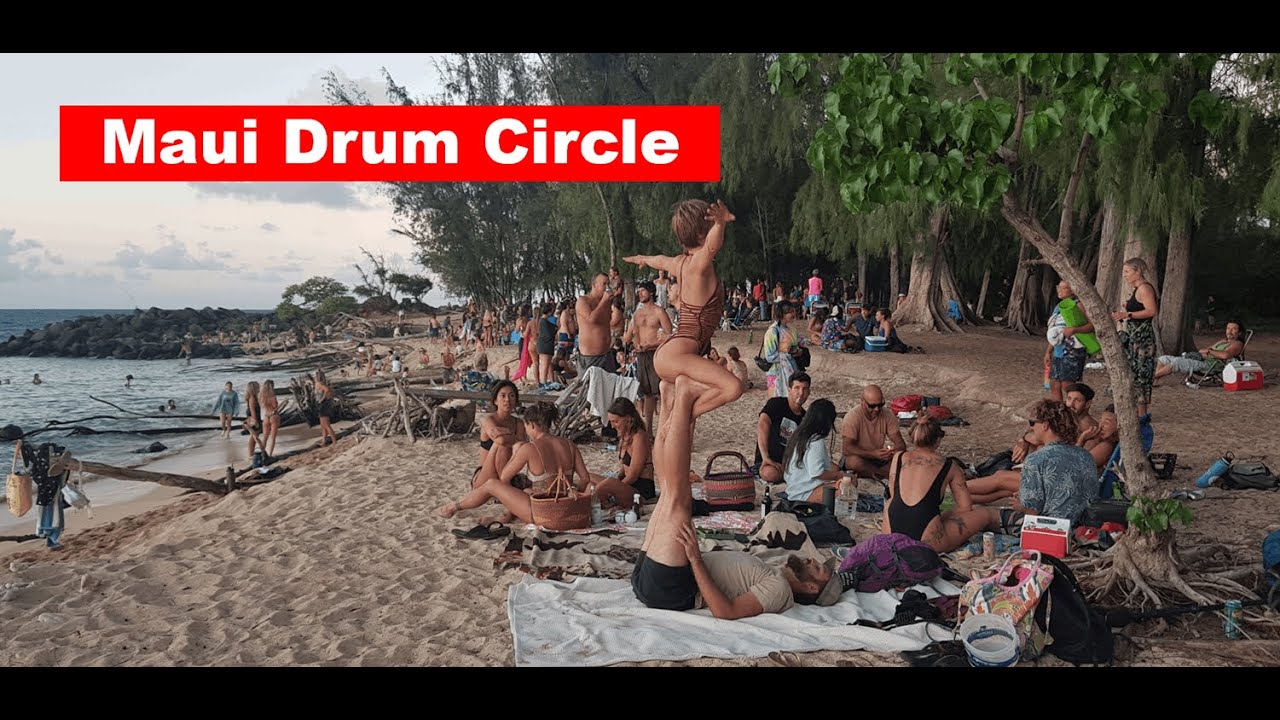A vibrant, full-color photograph captures a bustling beach scene under natural daylight, enclosed in a black border at the top and bottom of its horizontal frame. Central in the image’s upper left corner is a red banner with white text reading "Maui Drum Circle." Against a backdrop of sky and clouds, the center left unveils the ocean, while trampled sand populated with numerous footprints spans the lower left. The upper right brims with trees, and the lower right features an intriguing tree with an exposed root system. The beach is alive with activity, populated by people—primarily dressed in mid-century style bathing suits and casual clothes—enjoying the summer atmosphere. In the forefront, a bearded Caucasian man lies on a white, rumpled towel, lifting a woman in a gymnastic pose; she balances on his feet, her arms outstretched in a stylish bathing suit. Items like a purple object and bags scatter on the towel nearby. Additional details include picnic baskets and camper holders amidst the greenery, with circles of people socializing in the background, embodying a carefree 60s vibe. The beach's bumpy, footprint-laden surface adds to the dynamic, nostalgic scene.